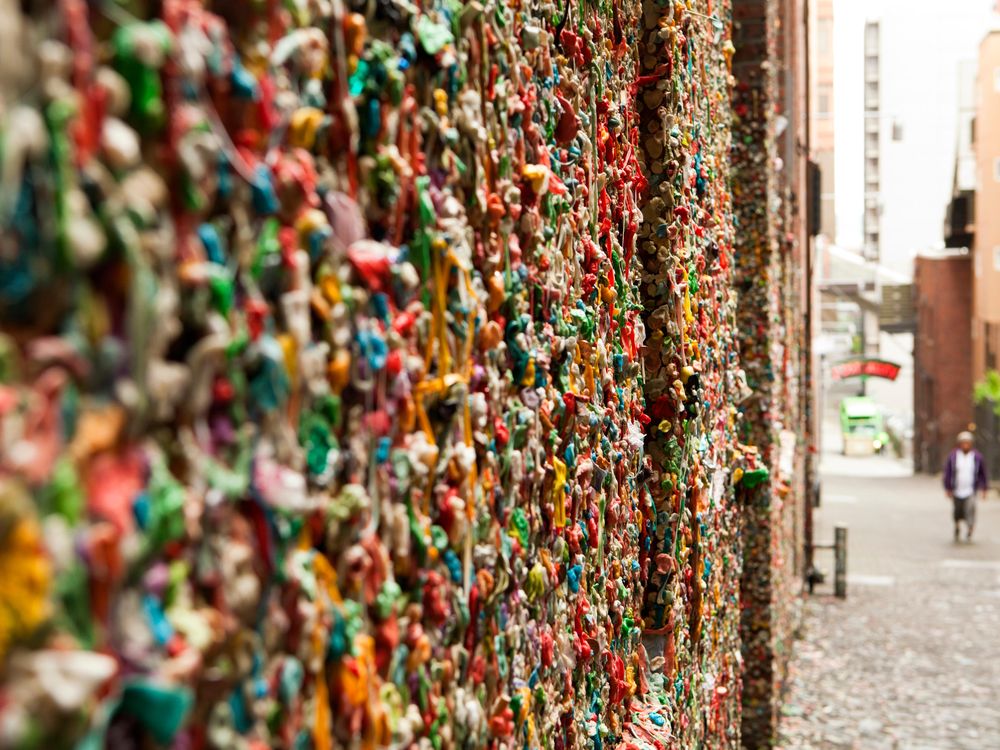The image showcases a vibrant and colorful street scene centered around an intriguing wall decorated with a dense array of hanging items. This wall, which forms part of a building, is adorned with what appear to be hundreds of thousands of tiny objects, including possible keychains, deflated balloons, and potentially strings of jewelry or beads. The objects drape across the wall in a kaleidoscope of colors, featuring hues of red, yellow, green, blue, purple, orange, and cream, creating a mesmerizing and bumpy texture. The close-up angle of the photo makes it difficult to identify each individual item distinctly, adding to the mystique. To the right side of the image, there is a glimpse of the street with regular brick buildings in the background, alongside a person dressed in a white t-shirt, purple coat, shorts, and a hat, walking under the sun's glare. The overall scene combines elements of urban life and vibrant artistry, capturing an eye-catching and colorful moment.